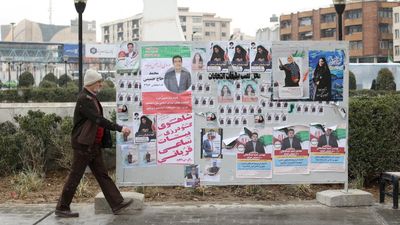This color photograph captures a man strolling down a wet sidewalk in a metropolitan city, indicated by the tall buildings and the distant elevated railway. The man, seen from his right profile, is dressed in a light-colored knit cap, a brown jacket, and brown pants, walking towards the right side of the frame. Dominating the scene is a large gray bulletin board mounted on two concrete blocks, filled with various posters. Among these, several feature images and text suggesting political campaigns or community events; one prominent poster showcases red Arabic writing on a white background, while another displays a sequence of photographs of a person. The posters, totaling at least five, are positioned in the middle and surrounded by smaller ones. To the right of the board, there is a bench, and the background includes hedges, a concrete wall, and two black lampposts flanking the scene. The wet sidewalk reflects the aftermath of a recent rain, adding a layer of ambiance to the urban streetscape.